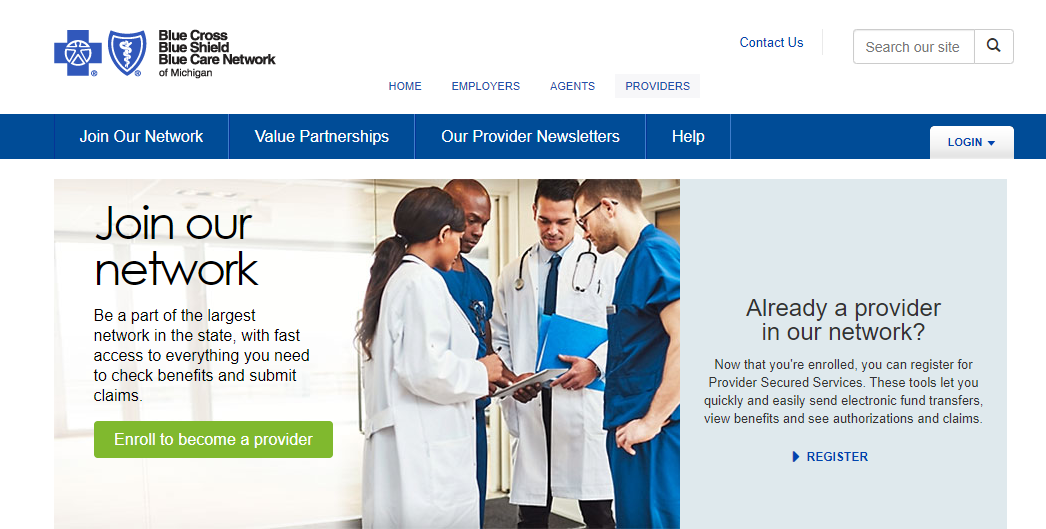Here is the cleaned-up and detailed caption:

---

This screenshot captures the homepage of the Blue Cross Blue Shield insurance website. In the top left corner, the Blue Cross Blue Shield logo is prominently displayed, featuring a blue cross with a circle and a star inside it, alongside a blue shield emblazoned with a snake icon. Adjacent to this, stacked phrases in black text read "Blue Cross Blue Shield" and "Blue Care Network of Michigan."

To the right of the logo, there's a navigation banner with links labeled "Home," "Employers," "Agents," and "Providers," with the "Providers" link currently selected. In the top right corner, accessible links include a "Contact Us" blue hyperlink and a "Search Our Site" search bar.

Below the primary navigation, a secondary blue banner lists options such as "Join Our Network," "Value Partnerships," "Our Provider," "New Sellers," and "Help," with a white-text "Login" dropdown menu positioned at the far right.

The main content area features an image of four medical professionals—three men and one woman—engaged in a discussion around a clipboard. The woman appears to be Hispanic, one man is African-American, and the remaining two men are Caucasian. 

To the left of this image, text invites users to "Join Our Network" and be part of the largest network in the state, highlighting benefits such as fast access to tools for checking benefits and submitting claims. Below this invitation is a green button labeled "Enroll to Become a Provider." 

To the right of the button, a message addresses existing providers, encouraging them to register for provider secured services. These tools enable quick and easy electronic fund transfers, benefit viewing, and claims authorizations. Below this message, there is a blue hyperlink titled "Register."

---